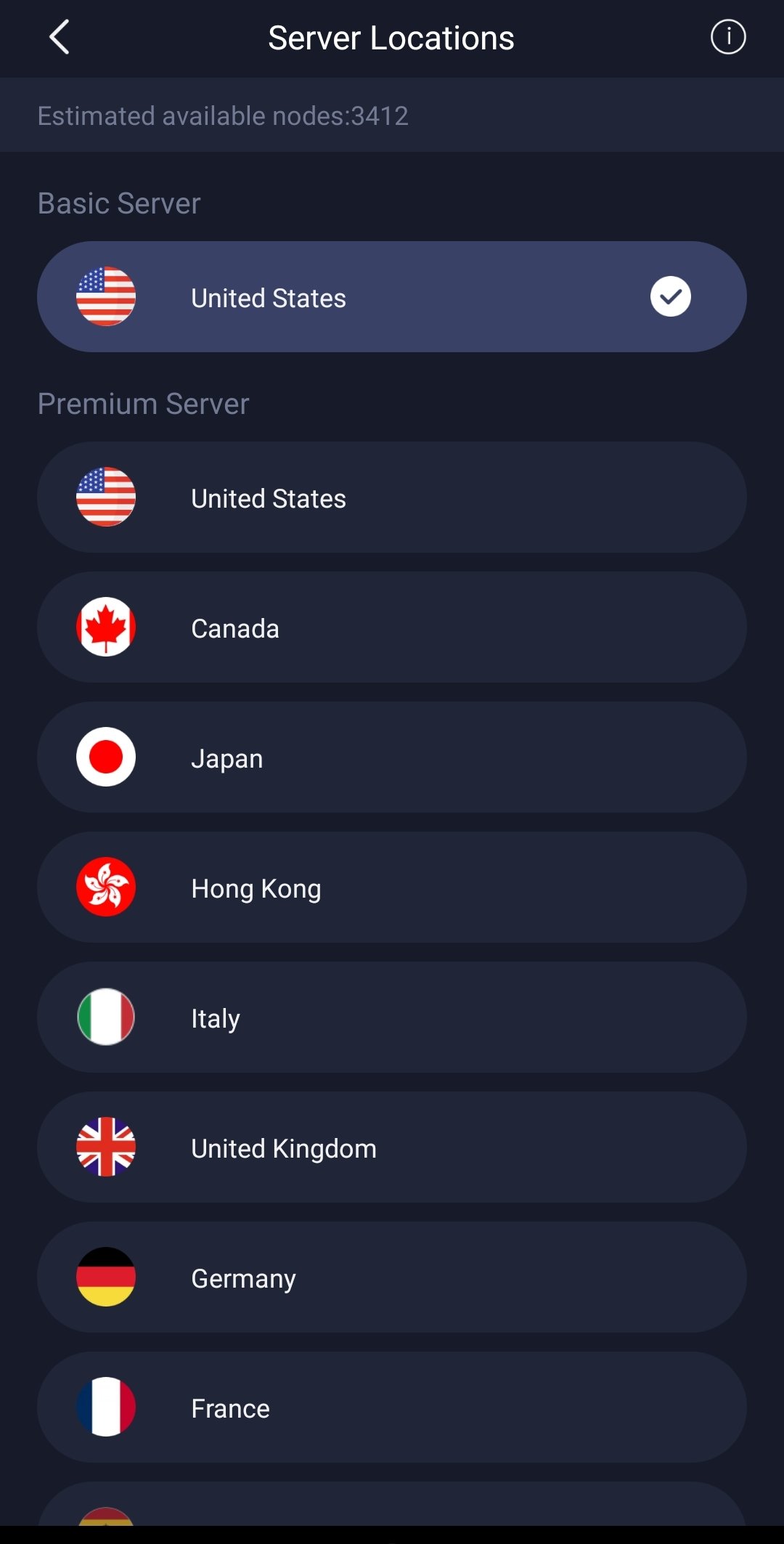Screenshot from a mobile phone displaying a section titled "Server Locations." The background is predominantly black, with a slightly lighter dark gray stripe running beneath the title. Centrally in the stripe, gray text reads "Estimated Available Nodes: 3412." 

Below this, the first section is labeled "Basic Server," featuring a United States flag next to the text "United States," accompanied by a checkmark, indicating selection.

The next section is labeled "Premium Server," listing various countries, each represented by their respective flags. The countries and their order are as follows:
1. United States
2. Canada
3. Japan
4. Hong Kong
5. Italy
6. United Kingdom
7. Germany
8. France

Each country is displayed within a dark gray oblong box, slightly lighter than the black background, with the country name and flag clearly visible.